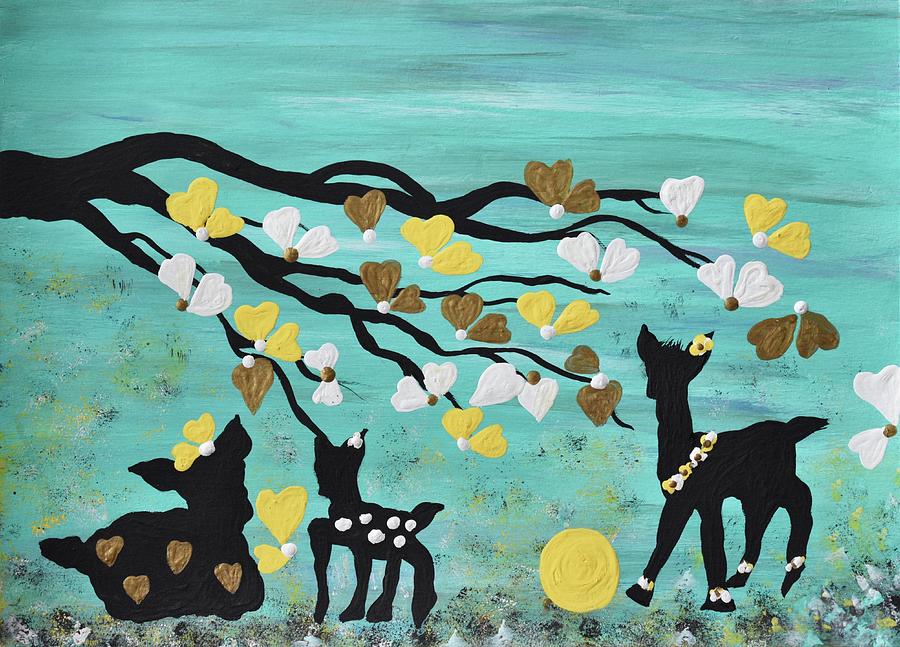This image is a detailed and textured painting on canvas with a captivating mix of colors and elements. The background is a wispy blend of turquoise, blue, and white, creating a dreamy, sky-like appearance. Anchoring the scene is a black silhouette of a tree branch that stretches from the upper left of the canvas, adorned with delicate flowers in shades of yellow, white, and brown, which resemble butterflies fluttering at the branch’s ends.

Below this branch are three black silhouette deer, each adorned with unique accents of color. The deer on the right stands gracefully with a small flower in its ear, a garland of yellow and white flowers around its neck, and white flowers around its hooves. The deer on the left is lying down and is distinguished by gold hearts on its body and yellow heart-shaped flowers on its head. A smaller deer stands in the middle, marked by white dots on its back.

These deer appear almost to float above a textured ground depicted with energetic black, white, and yellow brush strokes, giving the sense that the surface was poked and prodded with the brush to create an uneven terrain. Among these brush marks lies a yellow circle resembling a playful ball, seemingly at the ready should one of the deer decide to kick it. Altogether, the scene exudes a whimsical yet serene atmosphere, blending the ethereal with the playful.